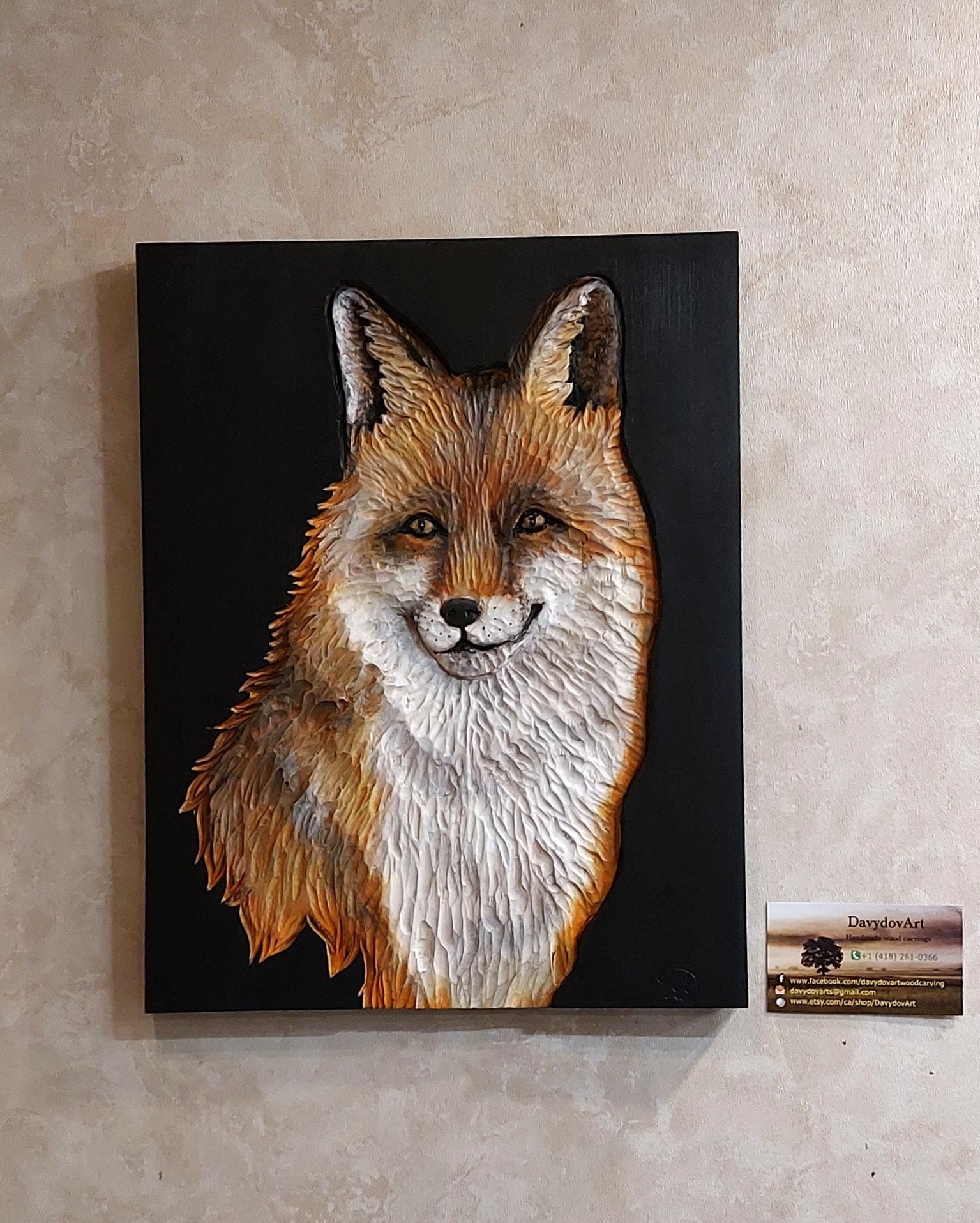In this detailed photographic image, an indoor setting reveals a striking canvas painting, prominently displayed on a textured, off-white to grayish gallery wall. The painting itself features a fox, executed with thick, almost 3D-like brush strokes, indicative of oil paint. The fox has a rich palette: brown fur with a black nose, pointed ears that are dark on the inside and whitish on the outside, golden eyes, a white chest, and an orange forehead. The image captures the fox in a cartoony yet detailed style, with its front face looking directly at the viewer, cropped around the belly and shoulder area. The canvas, hanging unframed against the wall, has a vertical orientation set against a black background that contrasts sharply with the wall's texture. To the right of the painting hangs a label that reads "Davidoff Art" along with a partially readable phone number, 415-241-0356, and an out-of-focus URL beginning with "www." Additionally, part of a ruler appears on the right, suggesting a way to measure the artwork.